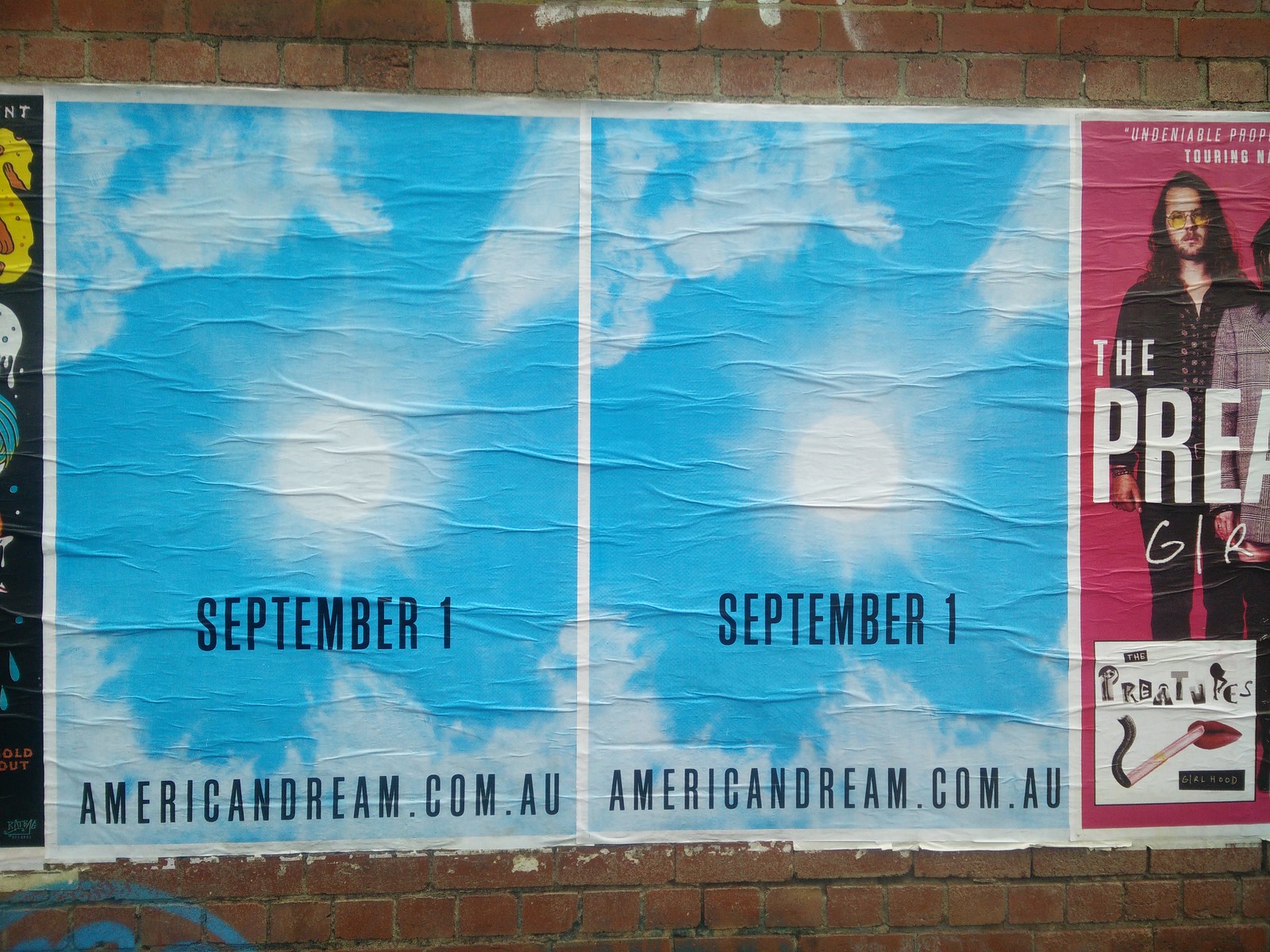This image features a large, thin material, reminiscent of a poster but of a different composition, adhered to a brick wall. The display consists of four visible panels. The far-left panel, only partially visible, showcases a yellow "S" with water droplets and the words "sold out." The central panels depict a serene blue sky with a blazing white sun at the center, bordered by fluffy white clouds. Beneath this idyllic scene, the text reads "September 1" followed by "americandream.com.au." The far-right panel reveals part of an image of a man dressed in black, with long hair, a beard, and a mustache. The man, who is white, also sports glasses with yellow-tinted lenses. The text on this panel begins with the word "undeniable" and includes the word "touring." At the bottom of this panel is an artistic rendering of a mouth holding a cigarette with some indistinct letters beside it.